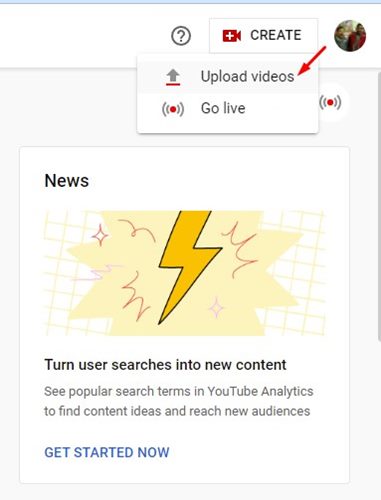This is an image of a partial screenshot, likely taken from a smartphone. At the top of the image, there is a light blue border running horizontally. Below this border, in the center, is a question mark enclosed in a circle. To its right, there is a rectangular box containing a red camera icon with a plus sign, followed by the word "create." 

Adjacent to this, there is a user profile image, and an arrow pointing left towards another rectangular box labeled "upload videos." Below this box, there is an arrow pointing up, accompanied by a red underline, and the text "go live" with a corresponding icon. To the right, outside of the box, there is another "go live" icon. The background in this section is light gray.

Further down, a square box is visible, containing the word "news" as its main header. Beneath this, there is a lightning bolt rendered in a cartoonish style, with a large star in the background indicating significance or impact. The background features gold squares with white centers, arranged at an angle.

Underneath this decorative element, the text reads "turn user searches into new content." Additional information pertaining to this statement is provided, followed by a "get started now" button located at the bottom left of the image.